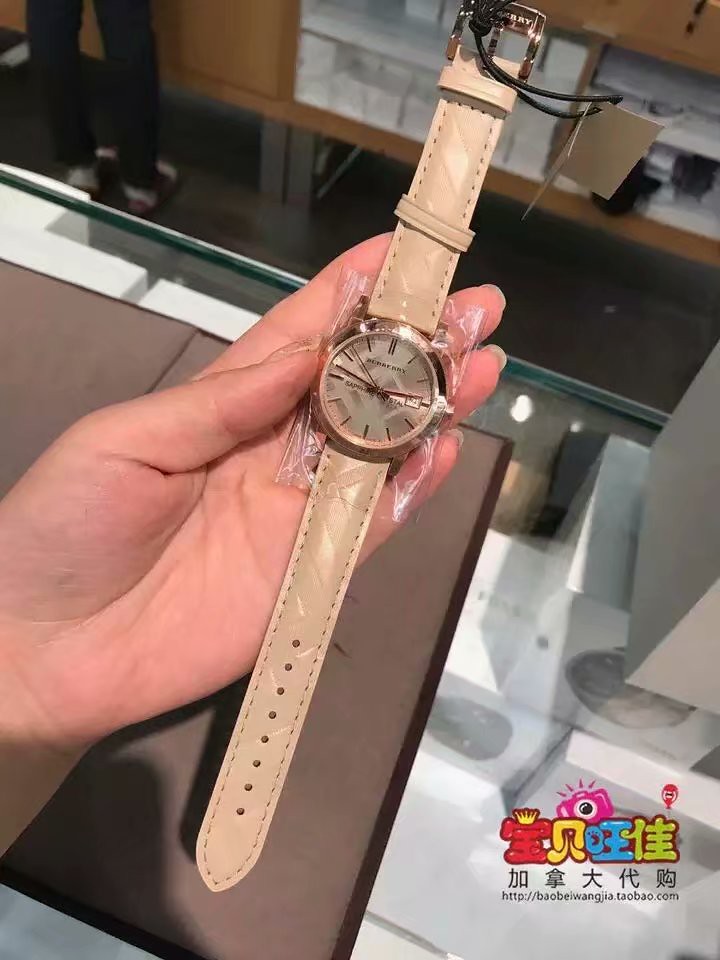This detailed image shows what appears to be a woman's hand, characterized by its narrow shape and elongated nail beds, holding a Burberry watch. The watch features a thin, light beige strap with multiple adjustment holes and a gold clasp inscribed with "Burberry" in light gold or beige lettering. The watch face, still wrapped in protective plastic, has a sleek design with only lines to mark the hours, and a background that shimmers between silver and copper tones. The scene appears to be set in a store or jeweler's shop, evidenced by a glass counter and various items in the background, including packaging that resembles printer paper and a white object possibly a fax machine with glasses on top of it. In the upper left corner, a pair of legs clad in tight jeans or black leggings is visible, wearing shoes that resemble bowling shoes or socks and sandals, with a distinctive red and white color pattern. At the bottom right of the image, there's a colorful logo with Chinese characters and the website "baobeiwangjia.taobao.com" in playful red, yellow, blue, and green letters, along with a pink camera icon. The photo likely serves as an advertisement, not only showcasing the watch but also emphasizing the brand and the purchasing platform.